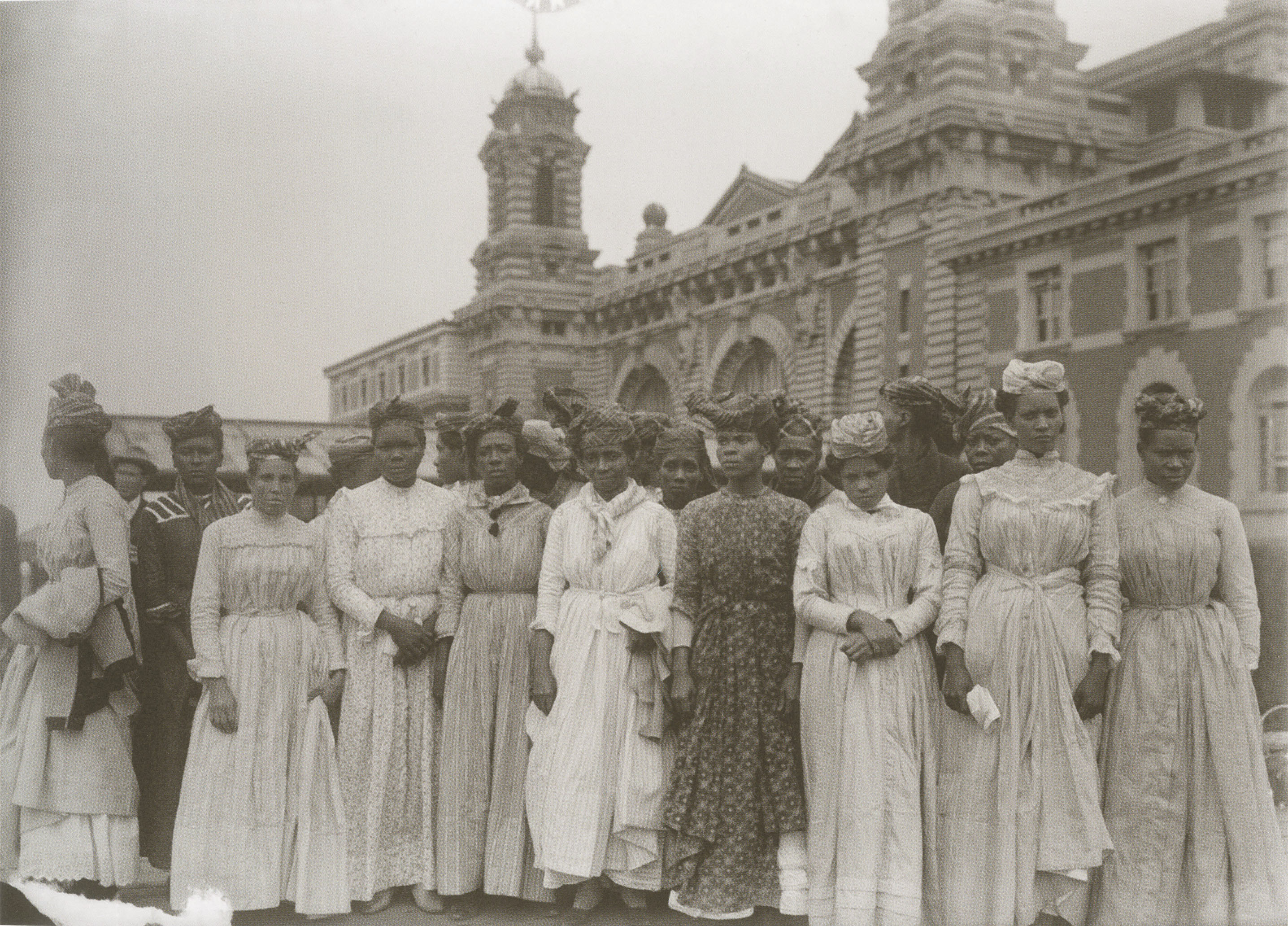This is a vintage black and white photo showcasing a large group of African women dressed in elegant European clothing, reminiscent of the 18th or 19th centuries. They are gathered in front of a grand, classic architectural hall, possibly a manor or mansion. The women, numbering around 20 to 30, are adorned in long dresses, primarily in black and white, with many of them sporting flowery hats on their heads. The detailed attire, which includes sleeves that mostly reach their wrists, appears to be their Sunday best, indicating a high-class status. Some of the women wear elaborate or floral-patterned dresses that stand out against the more monochromatic outfits. While it is difficult to determine if they are barefoot, their somber expressions are clear. In the background, a few gentlemen in traditional uniforms can be seen, adding to the historical context of this evocative photograph.